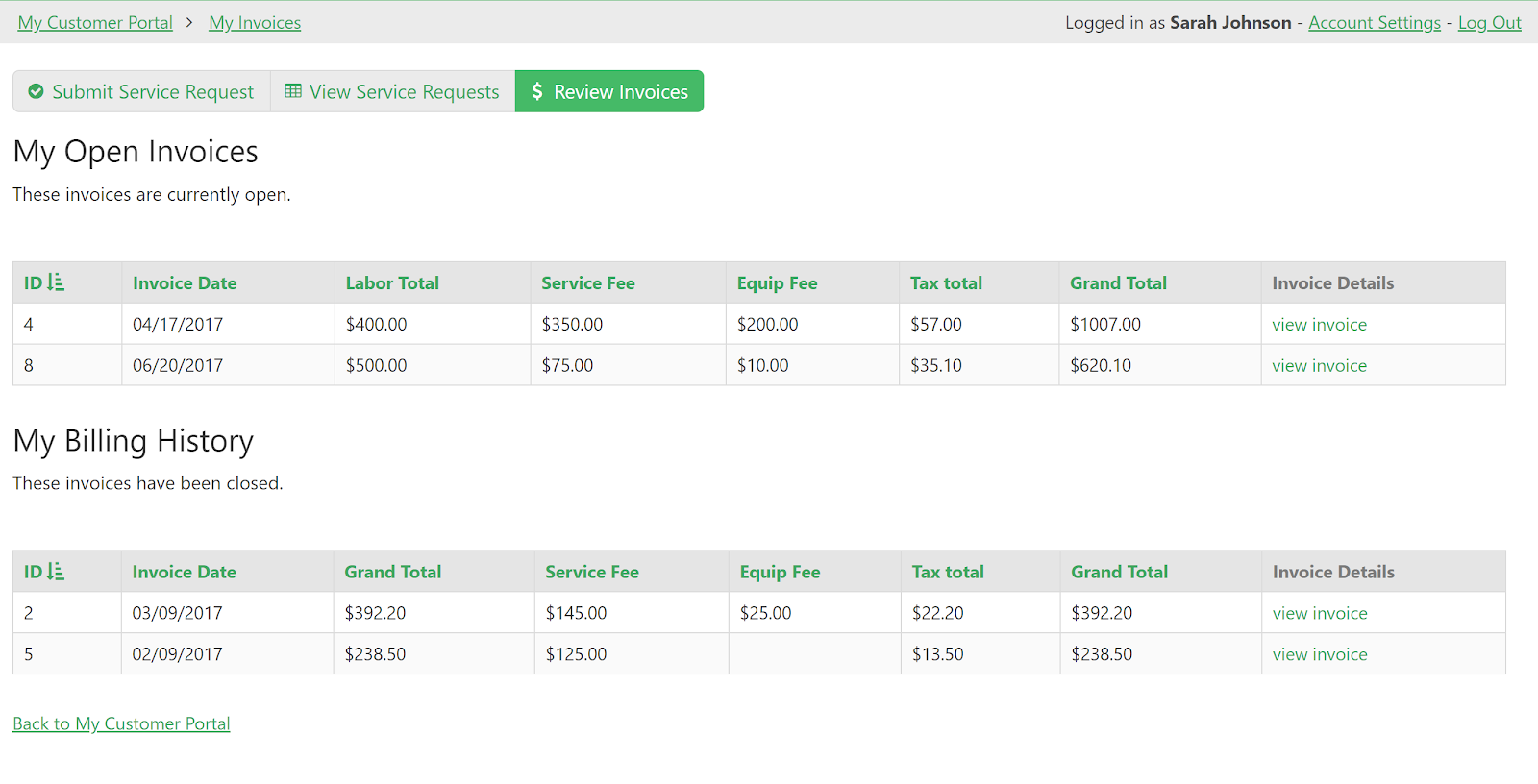### Detailed Caption:

The image features a user interface with a light blue background and several distinct sections, each providing important account information. At the top, in green letters and underlined, is the header "My Custom Portal." Directly to the right of the header is a right-facing arrow followed by the text "My Invoices," which is also underlined. Below this, the user is identified as "Logged in as: Sarah Johnson," accompanied by links to "Account Settings" and "Logout."

A prominent blue box below holds two sections: "Submit Service Request" with a small green circle and a check mark, and "View Service Request." Adjacent to this is a green box featuring a dollar sign and the text "Review Invoices."

The next section displays "My Open Invoices," with a subtitle stating "These invoices are currently open." Within this section is a blue box detailing invoice information with labels in green print: "ID," "Invoice Date," "Labor Total," "Service Fee," "Equip Fee," "Tax Total," "Grand Total," and "Invoice Details." Listed under this are two invoices:
1. **Invoice #4**
   - Date: April 17, 2017
   - Labor Total: $400
   - Service Fee: $350
   - Equipment Fee: $200
   - Tax Total: $57
   - Grand Total: $1,007
   - Option: View Invoice
2. **Invoice #8**
   - Date: June 20, 2017
   - Labor Total: $500
   - Service Fee: $75
   - Equipment Fee: $10
   - Tax Total: $35.10
   - Grand Total: $620.10
   - Option: View Invoice

The final section titled "My Billing History" shows "These invoices have been closed." It includes a blue box similar to the one used for open invoices, with labels in green print: "ID," "Invoice Date," "Grand Total," "Service Fee," "Equip Fee," "Tax Total," and "Invoice Details." Listed under this are two invoices:
1. **Invoice #2**
   - Date: March 9, 2017
   - Service Fee: $145
   - Equipment Fee: $25
   - Tax Total: $22
   - Grand Total: $392.20
   - Option: View Invoice
2. **Invoice #5**
   - Date: February 9, 2017
   - Service Fee: $125
   - Equipment Fee: None
   - Tax Total: $13.50
   - Grand Total: $238.50
   - Option: View Invoice

At the bottom of the image, there is a green and underlined text "Back to my customer portal."